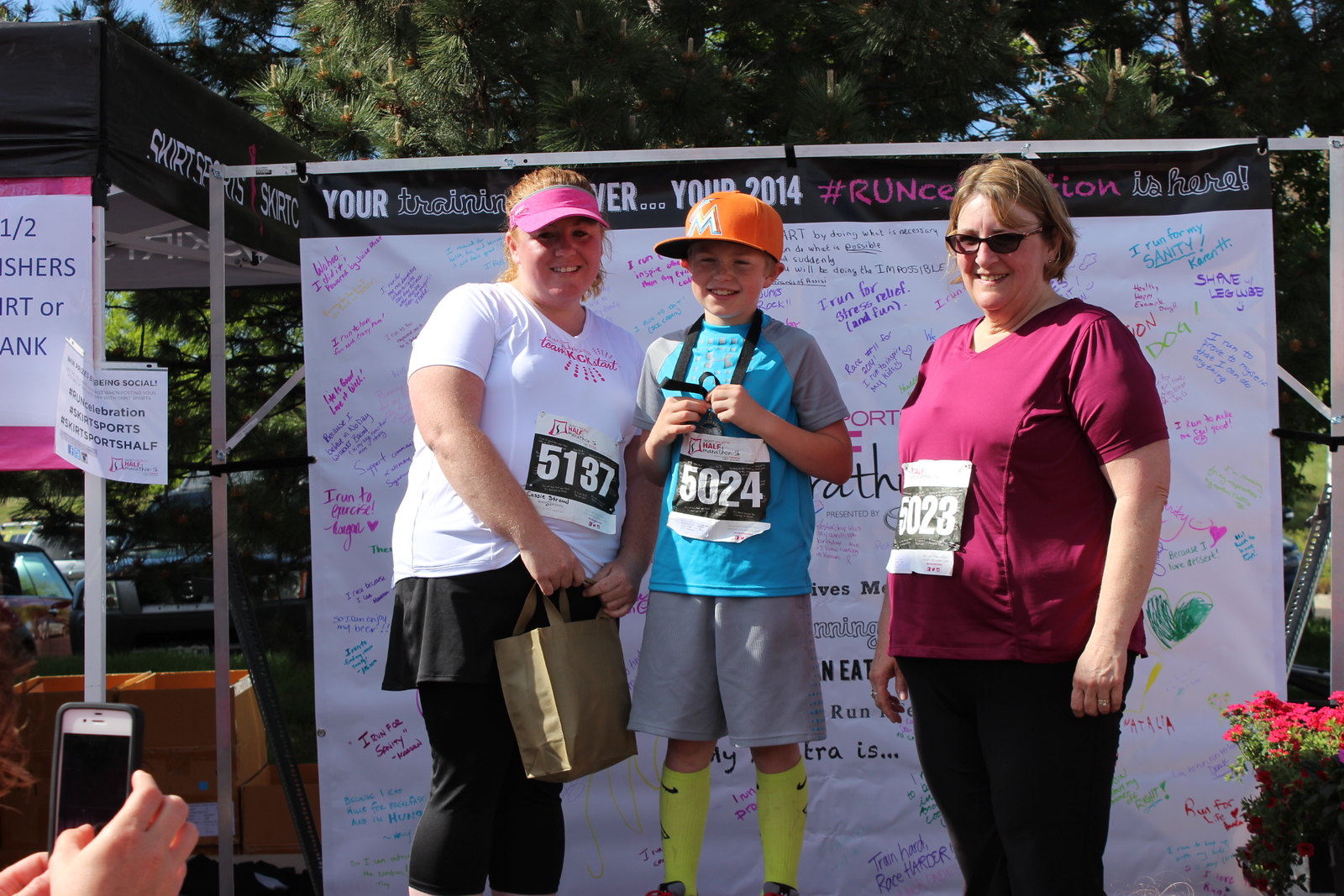In this outdoor photograph, three individuals stand proudly in front of a white banner covered with vibrant, multicolored signatures and the year "2014" prominently displayed at the top. The banner hangs from a silver rail, lending a celebratory feel to the scene. Centered on a pedestal is a school-aged boy, possibly around 13 years old, adorned in an orange hat, a blue-grey top, grey shorts, and knee-length lime green socks, numbered 5024 on his blue shirt. Flanking him are two women, both also wearing bib numbers, indicative of their participation in a competition, likely a race. The woman on the left sports a pink visor, a white T-shirt, black pants with a short black skirt overlay, and carries a tan bag. Her bib number reads 5137. On the right, the second woman, equipped with sunglasses, dons a dark purplish-red T-shirt and dark pants, her number 5023 visible. All three appear to be celebrating their achievements, captured in this rectangular, poster-like image that exudes the joy and camaraderie of the event.